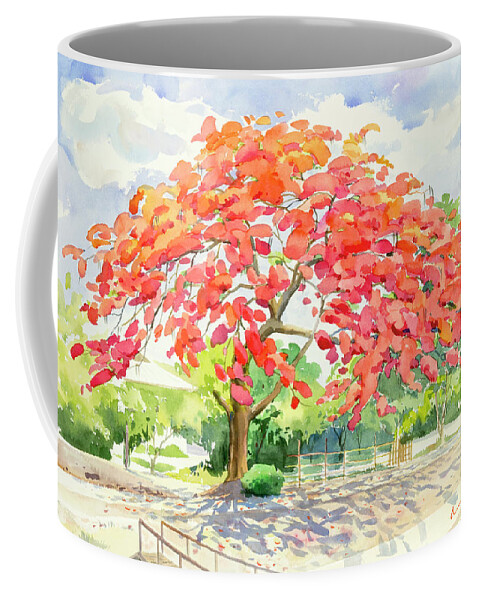This image features a white coffee mug with a light gray interior and a white handle on the left side, all set against a stark white background. The mug is adorned with a vivid color illustration. Dominating the scene on the mug is a tree with a brown trunk and branches topped with red, coral, and pink leaves. Accompanying this tree are smaller green shrubs at its base and some scattered leaves on the ground, suggesting an autumnal setting. The backdrop of this illustration includes a blue sky filled with fluffy white clouds and a distant fence line, leading to more green trees and a faint outline of a mountain. A narrow walkway with a mix of white and tan soil winds through the scenery, and shadows cast along the pathway take on a purplish hue, adding depth to the portrayal. The overall style is a blend of photographic realism and illustrative elements, making the image appear both lifelike and artistically rendered. The illustration wraps slightly around the mug, although not seamlessly. The crisp white background makes the mug and its detailed artwork appear as if floating.